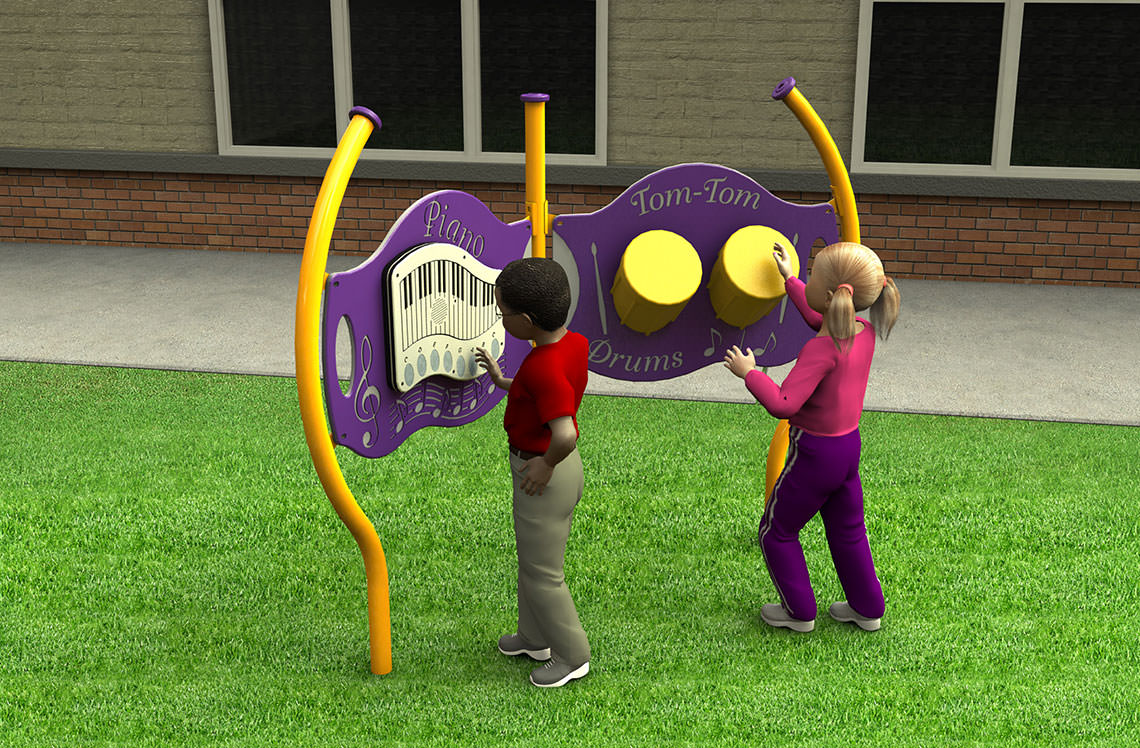This computer-generated, video game-like image depicts two animated children, a boy and a girl, from behind as they engage with a colorful playground contraption set on a grassy area. The scene is backed by a brick building with closed-window facades trimmed in white, adding an urban touch to the setting. The boy, identifiable by his dark brown hair, red t-shirt, and tan khaki pants, plays a two-dimensional toy piano. The girl, with blonde pigtails, a pink shirt, and dark purple pants, interacts with a tom-tom drum set. The playground structure features three yellow poles and curved purple panels, designed with "piano" inscribed on the left panel and "tom-tom" on the right, enhancing the playful learning environment. The vibrant contrast and animated depictions suggest this image belongs to a video game or digital illustration, emphasizing the imaginative and interactive atmosphere.